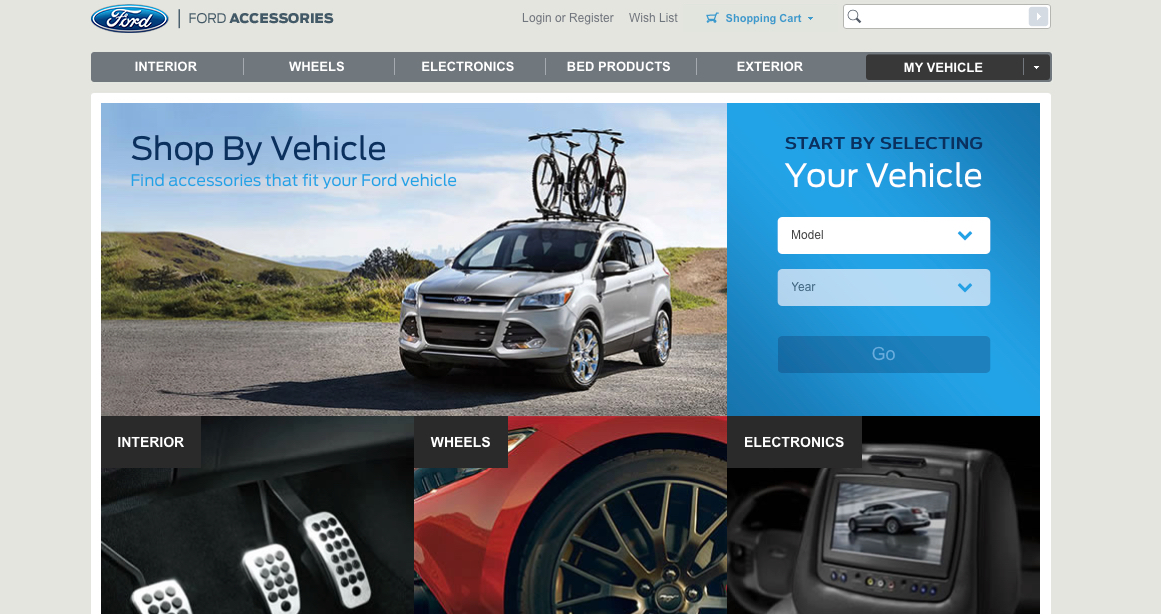The webpage displayed is an official Ford accessories page. The top right corner features the iconic blue and white Ford logo, spelled "F-O-R-D." To the right of the logo, "Ford Access" is inscribed. Adjacent to this are links for "Login or Register," "Wishlist," "Shopping Cart," and a search bar.

Below these links is a grey navigation bar housing several white text tabs: "Interior," "Wheels," "Electronics," "Bed Products," "Exterior," and "My Vehicle," the latter of which is currently selected. 

In the section beneath the navigation bar, an area with a blue background prompts users to begin by selecting their vehicle's model and year from dropdown menus, alongside a "Go" button. To the left of this section is an image of a silver-grey Ford vehicle equipped with two bicycles mounted on the roof. Above this image, the text reads, "Shop by Vehicle. Find accessories that fit your vehicle."

At the bottom of the page are categorized sections. Starting from the bottom left, the "Interior" category is represented by an image of three pedals: brake, clutch, and accelerator. The "Wheels" section showcases a black-rimmed wheel with a black tire mounted on a red Ford Mustang, displaying the Ford Mustang logo on the wheel cap. The "Electronics" category on the bottom right features a picture of a vehicle's dashboard.